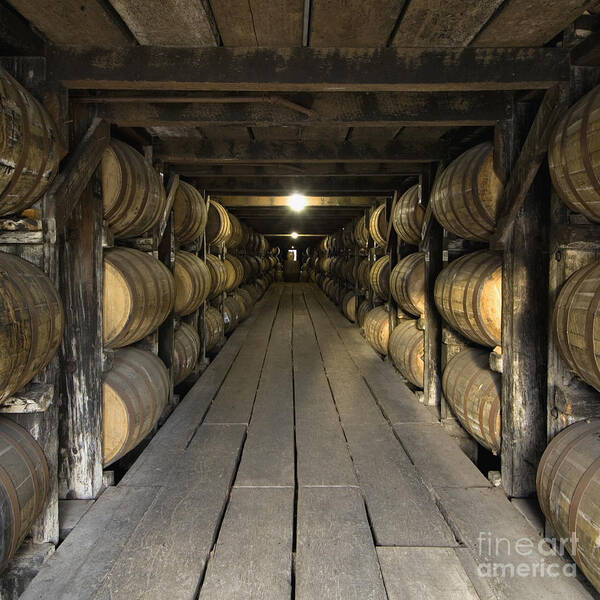The image depicts a dimly-lit, underground cellar resembling a storeroom or cave, adorned entirely in wood—from the floor to the ceiling and the supporting beams. The environment is rustic with rough, beamed ceilings and wooden planks forming a central walkway that stretches into the background. On either side of this walkway are two long rows of barrels, stacked three high and secured with metal rings. Each barrel shows signs of wear with a patina and some dirt, suggesting they have been in use for an extended period. The barrels could contain wine, whiskey, or beer, though their specific contents are not visible. Overhead, faint lights provide just enough illumination for the space, casting shadows that accentuate the earthy, varying shades of brown throughout the room. In the lower right corner of the image, there is a text label that reads, "Fine Art America." The overall atmosphere is one of aged craftsmanship, steeped in a rich history of fermentation and storage.